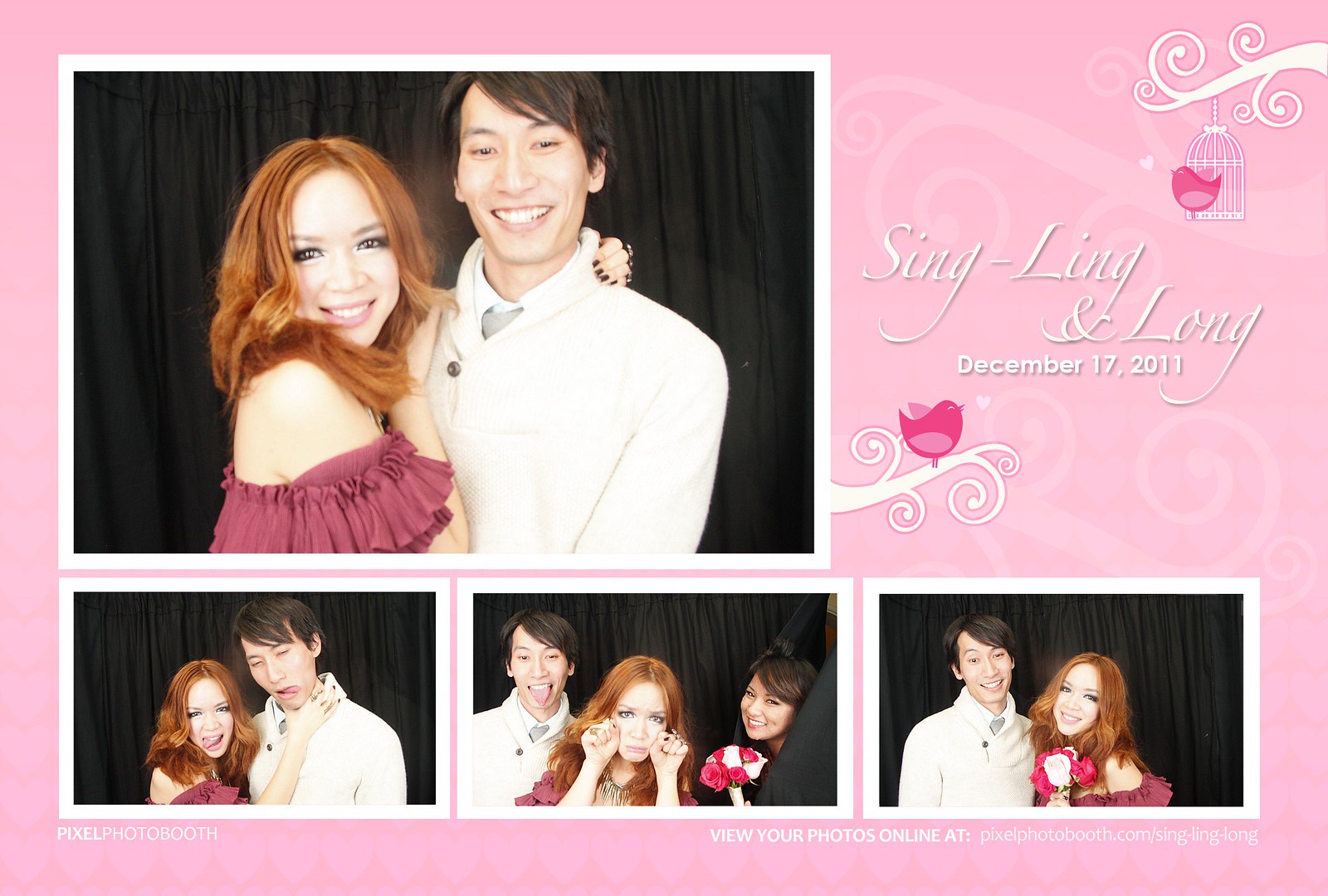This image is a detailed announcement card with a pink, slightly textured background. At the top, in stylized white font, it reads "Sing-Ling and Long, December 17, 2011." The design features a large central photograph of a young Asian couple, possibly at their prom or wedding. The man is on the right, donning a white suit with medium-length black hair combed over to his left eye, smiling warmly. The woman, on the left, has long red hair, a shoulder-exposing purple-red dress, and she’s smiling forward with her right hand on the man's shoulder and her left arm around his back. Behind them is a black curtain. Beneath this main photo, three smaller photos are arranged left to right. The first shows the same couple making silly faces, with the woman pretending to choke the man who has his tongue out. The middle photo includes another woman holding flowers, standing between the couple, and pretending to cry. The rightmost photo shows the couple smiling again, this time with the man on the left and the woman on the right. Additional decorative elements include a white tree limb drawing with a red flower at the top right border and another limb with a hanging cage and a red bird at the bottom right. There’s some faint white writing at the card's bottom, under the last two pictures, which isn’t fully legible.